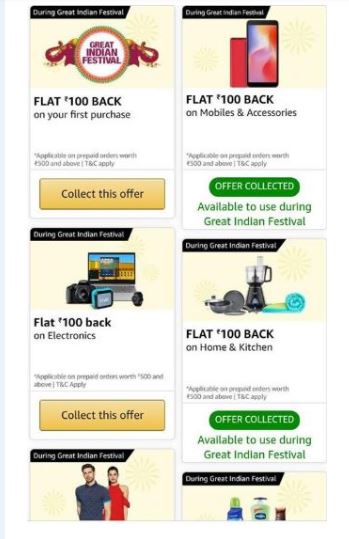The image displays a series of promotional offers linked to the Great Indian Festival event, showcased in six vertical rectangular panels. The offers are tacky and vibrant, sporting a variety of colors, including red, blue, purple, yellow, gold, green, turquoise, black, gray, and white.

1. **Top-left Offer:**
   - **Description:** "Flat ₹100 Back on Your First Purchase"
   - **Details:** Promoted during the Great Indian Festival
   - **Action Button:** Yellow "Collect this Offer"

2. **Top-right Offer:**
   - **Description:** "Flat ₹100 Back on Mobiles and Accessories"
   - **Details:** Available to use during the Great Indian Festival
   - **Action Button:** Green "Offer Collected"

3. **Middle-left Offer:**
   - **Description:** "Flat ₹100 Back on Electronics"
   - **Details:** Promoted during the Great Indian Festival
   - **Action Button:** Gold "Collect this Offer"

4. **Middle-right Offer:**
   - **Description:** "Flat ₹100 Back on Home and Kitchen"
   - **Details:** Available to use during the Great Indian Festival
   - **Action Button:** Green "Offer Collected"

To the far right of the image, only partial views of two additional offers are visible, suggesting continuity with the offers related to the Great Indian Festival. The abundance of colors and the repeated festival branding highlight the grand and celebratory nature of the promotions.